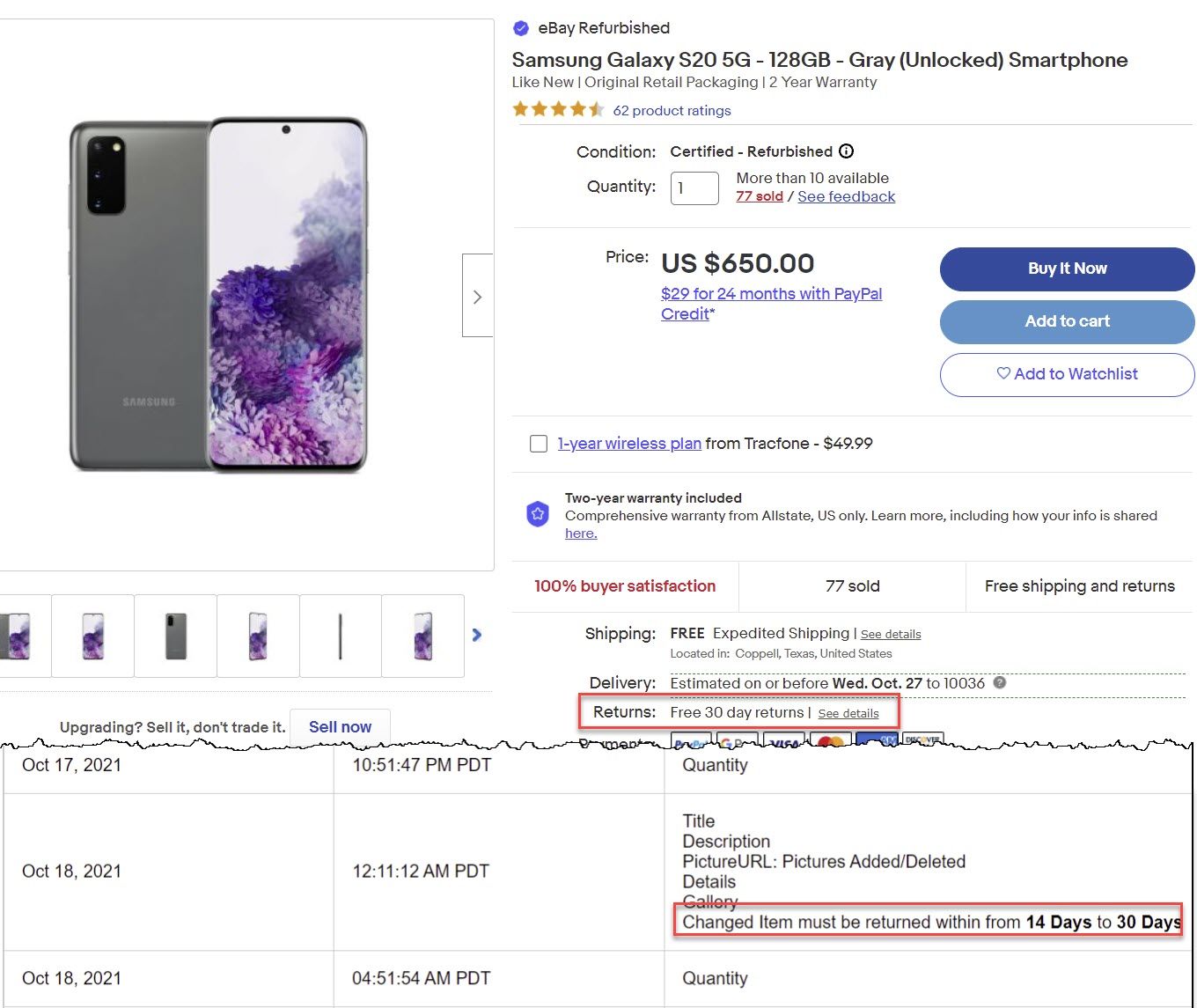The image depicts a detailed listing for purchasing a gray Samsung Galaxy S25G (128GB) unlocked smartphone on eBay. In the top left corner, there's an image of the phone front view against a white and purple background. Adjacent to this on the right is a purple check mark with "eBay refurbished" written beside it, and below it, "Samsung Galaxy S25G-128GB-Gray Unlocked Smartphone" is printed in black.

The listing highlights that the phone is like-new, packaged in original retail packaging, and comes with a two-year warranty. It boasts a four-and-a-half star rating out of five, based on sixty-two product ratings, with golden stars. The condition is certified refurbished, and the listing shows that there is a quantity of one available, with more than 10 units available and 77 units already sold.

Further details include a "See feedback" link, a price of $650, and options to "Buy Now," "Add to Cart," or "Add to Wishlist." Financing is offered at $29 for 24 months through PayPal Credit. Additionally, there's a square featuring a one-year wireless plan from TracFone for $49.99. The listing includes a comprehensive two-year warranty from Allstate, limited to the US, with a clickable link to learn more about privacy information. 

Highlighted features include 100% buyer satisfaction, free shipping, and expedited shipping from Coppell, Texas, with an estimated delivery date on or before Wednesday, October 27th, to ZIP code 10036. The return policy allows for free returns within 30 days, detailed within a red rectangle.

To the left, multiple images of the cell phone are displayed in small boxes showing different angles. Below, an option to upgrade your device with the message "sell it, don't trade it" and a "Sell Now" button is present. The bottom of the screen exhibits a cut piece of paper appearance, showing three boxes in three columns. Information tags with timestamps, such as October 17th, 2021, 10:51:47 PM PDT, October 18th, 2021, 12:11:12 AM PDT, and October 18th, 2021, 0-41-51-54 AM PDT indicate various updates and quality checks. These elements are within a red box stating the item must be returned within a 14- to 30-day window.